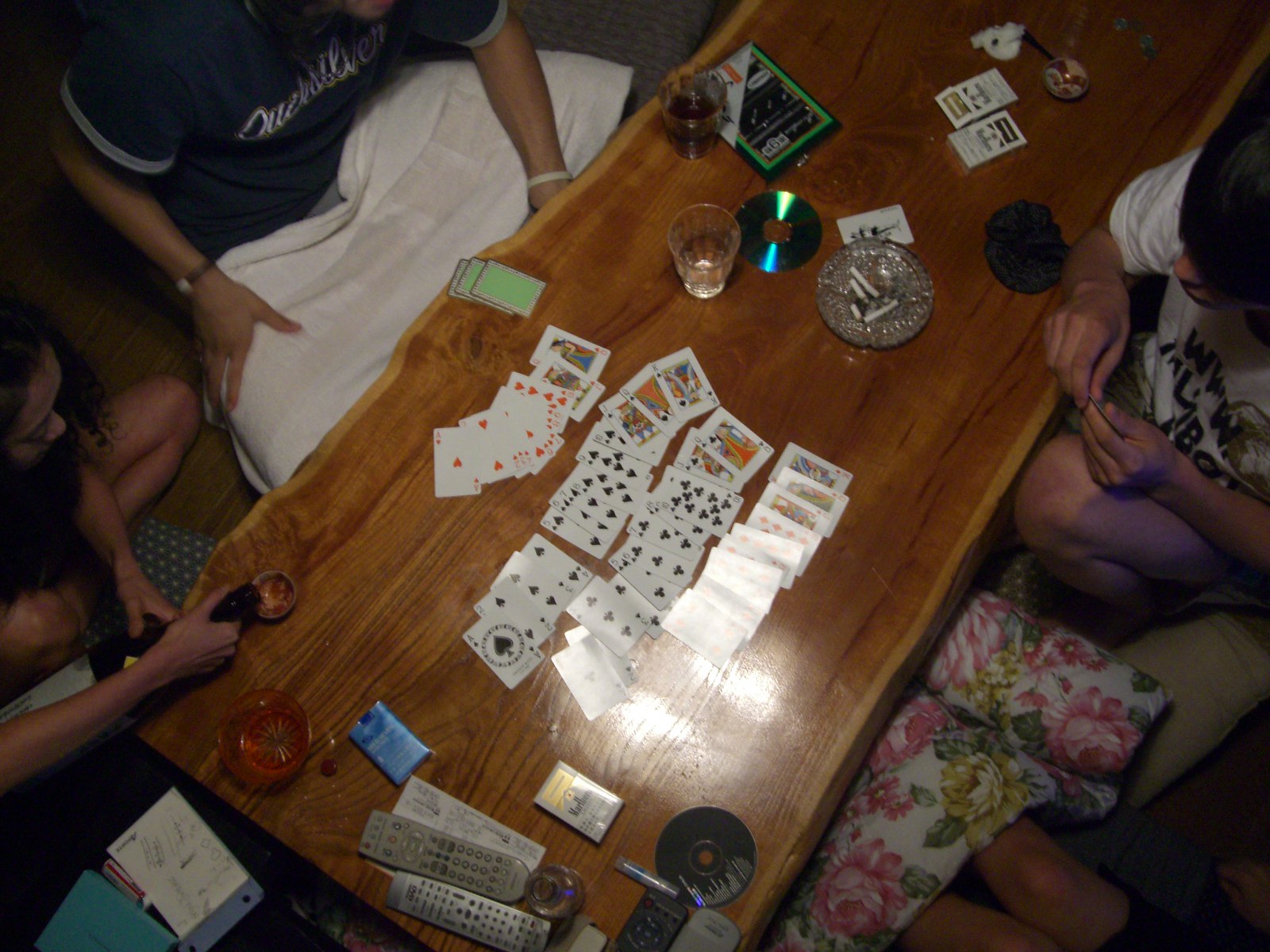In the image, a lively scene unfolds with several individuals engrossed in a card game around a table strewn with various items. On the left side of the image, we see two people. The person at the top left is wearing a blue short sleeve t-shirt, with a white towel draped across their legs, obscuring their pants or shorts. They have a yellow bracelet on their left wrist and a wristwatch with a brown band on their right wrist. To their right sits a woman with dark curly hair, dressed in shorts and a short sleeve t-shirt. She is in the act of pouring what appears to be wine into a cup. Next to her, a red plastic cup is visible alongside a blue pack of cigarettes.

Further to the right on the table, there is a collection of cream and dark tan colored TV remotes, another white pack of Marlboro cigarettes with a gold label at the top, and a dark gray compact disc. Spread out across the table are numerous playing cards, arranged face up, featuring hearts, spades, clubs, and diamonds in neat rows. An ashtray with cigarettes lies to the right of the cards, amidst more cigarette packs. Another CD is visible, this one turned upside down, alongside a couple of cups containing drinks.

On the far right of the table, two more individuals are partially visible. One person's legs are peeking into the frame, while the other person, dressed in a white short sleeve shirt, is seated with their gender indeterminate from the given vantage. The mood of the scene is casual and convivial, punctuated by the scattered items and the engaged expressions of the card players.